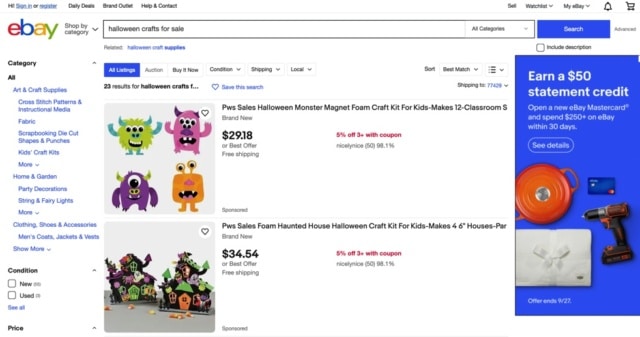This image features a detailed screenshot of the eBay website. The interface prominently displays the recognizable eBay logo situated at the top left corner. Aligned above the logo are multiple navigational links such as "Sign In," "Daily Deals," "Brand Outlet," "Help & Contact," indicative of user account access and customer service options. On the right-hand side of the top navigation bar, additional options include "Sell," "Watch List," "My eBay," alongside icons for notifications and the shopping cart.

Centrally located, the second row features a prominent search box where a query for "Halloween crafts for sale" has been entered. Positioned to the right of this search bar is another eBay logo, with adjacent dropdown menus for browsing categories, and a "Search" button followed by an "Advanced" search option.

The left sidebar showcases a categorized column where users can navigate through eBay's diverse product categories, starting with "All Categories." Visible categories include "Art and Crafts," "Home and Garden," and "Clothing, Shoes & Accessories," each with subcategories like "Cross Stitch Patterns" and "Fabric" under "Arts and Crafts."

The page displays results for the searched term "Halloween crafts for sale." Featured items include a "Halloween Monster Magnet" designed for children and a "Sales PWS Foam Haunted House Halloween Craft Kit." An additional ad promoting the eBay MasterCard is visible on the right side of the page.

Overall, the screenshot provides a comprehensive view of eBay's search functionality, user navigation options, and a glimpse into specific Halloween-themed product listings.